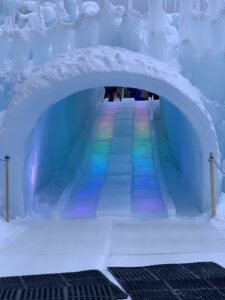This photograph captures the enchanting entrance of an ice cave or igloo-like structure, shaped as a giant archway made entirely of snow and ice, with the perspective of someone looking up from the bottom. The ice cave features a central double slide, designed with a distinct middle barrier, and bathed in rainbow colors. The vibrant hues of purple, dark blue, light blue, green, yellow, orange, and red illuminate the slide, possibly from colored lights embedded underneath or delicately crafted snow. On either side of the entrance, sleek poles stand symmetrically, possibly indicating the way in. The slide appears solid and well-constructed, leading up to a snow platform. Above the archway, various snow figures are sculpted, adding an artistic touch. At the bottom, two black rectangular mats are prominently placed, likely for the entrance. The background of the image is dark, enhancing the vivid colors of the slide and the mystical ambiance of the scene.